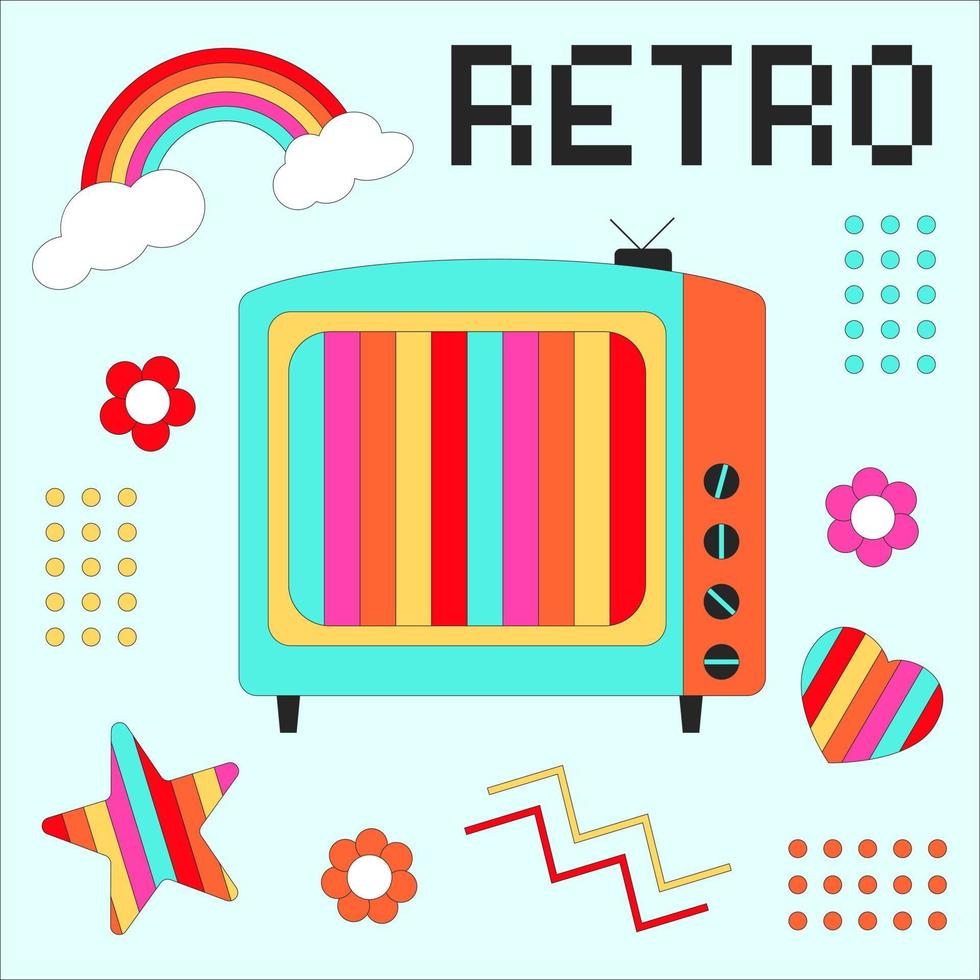This square, cartoon-style image features a retro TV at its center, characterized by a light blue front and orange sides fitted with four black dials adorned with blue stripes. The TV, topped with classic bunny ear antennas, displays vertical stripes in blue, pink, orange, yellow, and red. Above the TV, the word "RETRO" appears in a video game-like font, against a light blue background. In the top left corner, a rainbow with red, orange, yellow, green, and blue stripes is flanked by small clouds. Surrounding the TV are various whimsical elements: rows of light blue dots, pink flowers with white centers, a heart with rainbow stripes, orange flowers, red and yellow squiggly lines, a multicolored star, additional yellow and orange dots, and a small red flower.